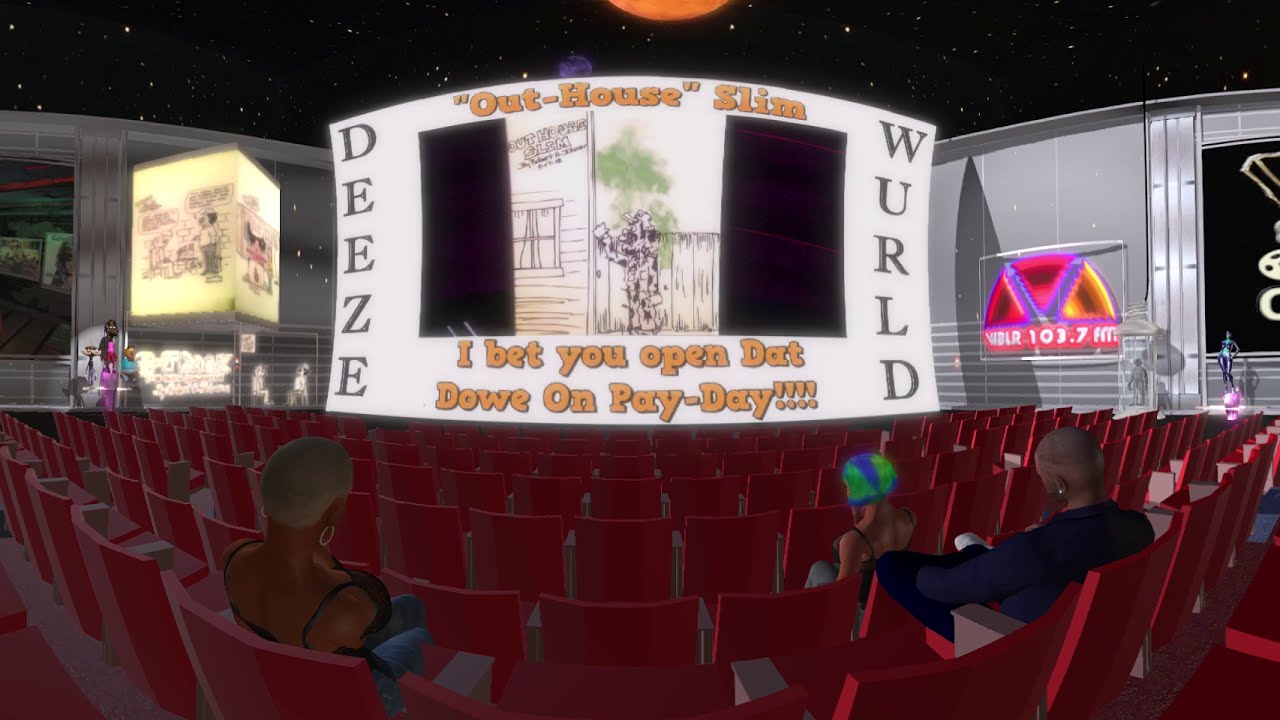The image is a horizontally oriented, digitally simulated auditorium scene viewed from the back with a distinct fish-eye effect that causes the scene to bend towards the center bottom. Rows of red chairs, sparsely populated with only a few individuals facing away from the viewer, fill the foreground. At the front of the auditorium, a large, curved, white billboard is prominently displayed, resembling a stage backdrop. The billboard features the vertically aligned words "D.E.E.Z." in large black letters on the left side and "W.U.R.L.D." in similarly large black letters on the right side. In the center of the billboard is an indistinct drawing, flanked by gold writing at the top and bottom edges that reads "Outhouse Slim" and "I Bet You Opened That Dough on Payday". Additional images appear on either side of the billboard, enhancing the digital simulation of the auditorium.